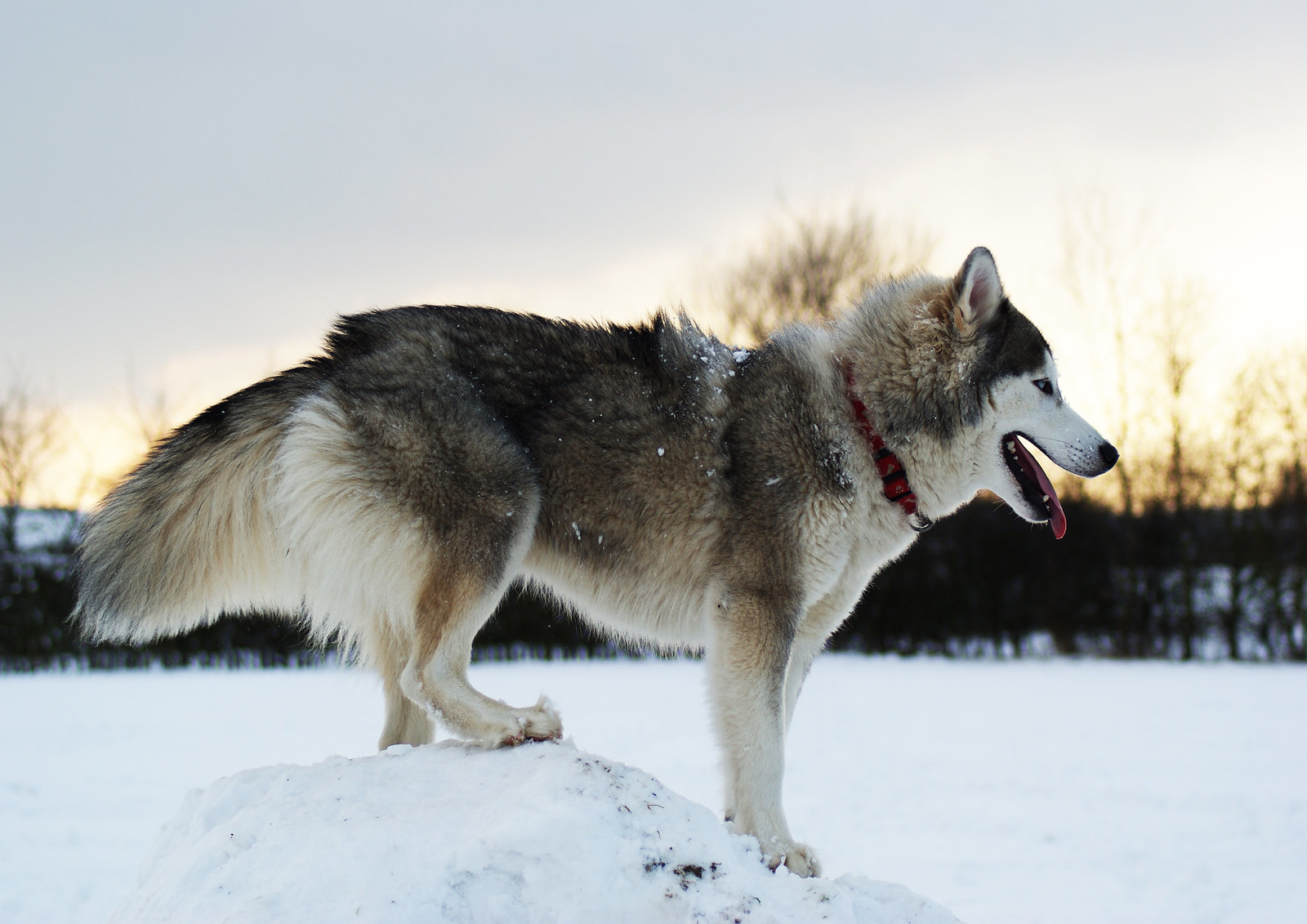On a cold winter afternoon, beneath a gray-blue sky with the sun setting low, a happy Alaskan Husky stands proudly on a mound of snow. His thick, fluffy fur features a striking blend of colors: white underneath, tan on his sides, and a darker shade along his top, with a white muzzle and face contrasting against his dark forehead and ears. The dog's pink tongue peeks out from his open mouth, and he wears a red and black collar around his neck. His bright blue eyes are focused elsewhere as he enjoys the snowy landscape. Bare, leafless trees frame the background, emphasizing the chilly, serene atmosphere of the day.